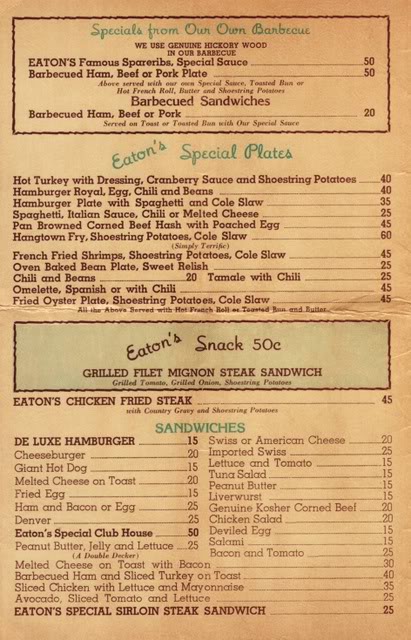A vertically oriented, long rectangular menu with predominantly black writing and accents of blue text. The centerpiece of the menu features a large rectangular blue panel with black writing, prominently announcing "Specials From Our Barbecue," and emphasizing the use of genuine hickory wood in their barbecue preparation. Among the offerings listed, Eaton's Famous Spare Ribs with special sauce are priced at 50 cents. Barbecued plates featuring ham, beef, or pork are likewise 50 cents each, while barbecue sandwiches with ham, beef, or pork are available for 20 cents.

The menu also highlights several special plates: Eaton's Special Plates include a hot turkey dish with dressing, cranberry sauce, and shoestring potatoes for 40 cents. Other hearty options include a Hamburger Royal with egg, cheese, and beans for 40 cents, a Hamburger Plate served alongside spaghetti and coleslaw for 35 cents, and Spaghetti adorned with Italian sauce, chili, and melted cheese for 25 cents. 

Additionally, the menu offers Pan-Browned Corned Beef Hash with a poached egg for 45 cents. Overall, the menu reflects remarkably low prices, prompting curiosity about the era from which it originates.